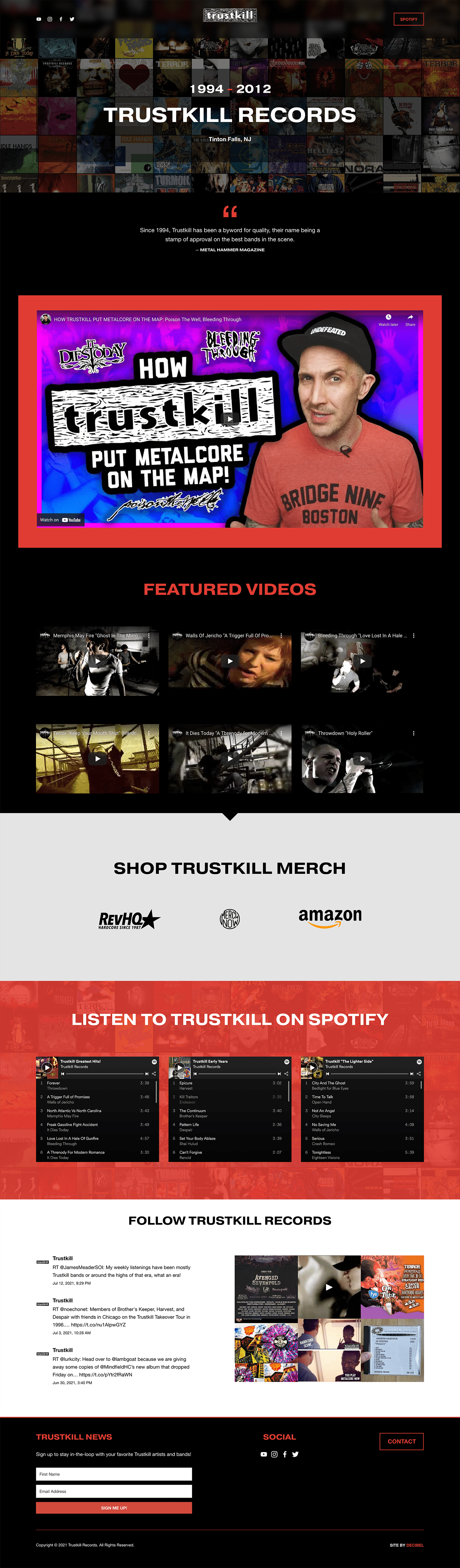A screenshot of a website featuring a distinctive red and black background. The image has a slightly blurry appearance. At the top of the screen, a man is visible alongside a long banner. The top of the page displays a logo reading "Traskill" in white text, set against a background resembling old TV static.

In the top left corner, there are social media icons for YouTube, Instagram (appearing as a TV screen logo), Facebook, and Twitter. The top right corner features a Spotify icon with a red outline and red text. 

Central to the top of the page, it reads, "1994-2012 Traskill Records, Tintin Falls, New Jersey," indicating this is for a now-defunct record company. Beneath this, there's a declaration: "Since 1994, Traskill has been a byword for quality, their name being a stamp of approval on the best bands in the cities," attributed to Metal Hammer Magazine.

In the middle of the page, there is a YouTube video link titled "How Traskill put Metalcore on the map." To the right of the video, a man is seen wearing a red shirt and a black hat.